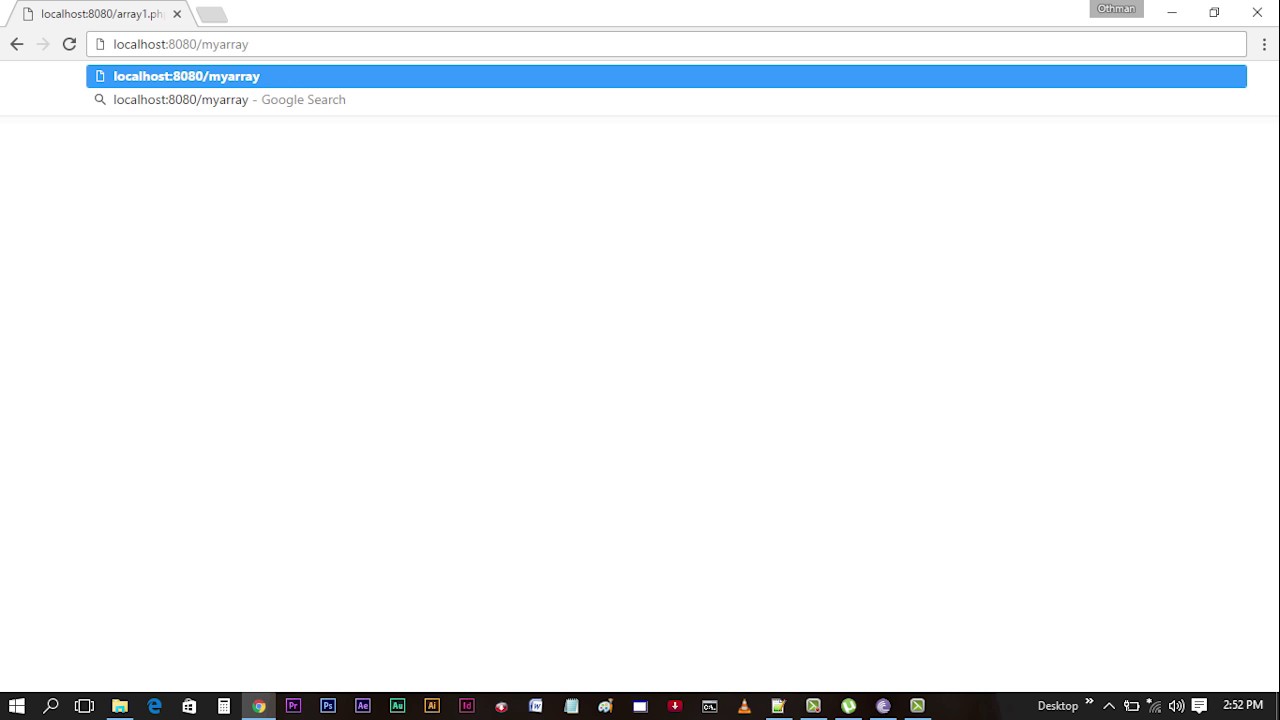The image shows a computer screen displaying a web browser in Windows OS. The URL bar reads "localhost:8080/myarray." Below the URL bar, a grey tab is visible. To the left of the tab, there is a back button, and to the right, a faded-out forward arrow, indicating that advancing to the next page isn't possible. The refresh button is next, followed by the URL input field where users can type or click web addresses. 

Highlighted in blue in the URL bar is "localhost:8080/myarray". Below this, there is a Google search option. In the top-right corner, there are window control buttons: minimize, maximize (or two squares for viewing two pages simultaneously), and close.

At the bottom of the screen, typical Windows UI elements are present. The bottom-left corner has the Start menu icon, search bar, Internet Explorer icon, and a file folder icon. The system tray at the bottom-right shows the battery being charged, volume control, and the current time, which is 2:52 PM. The taskbar displays several application icons, including Google Chrome, suggesting that it is currently active.